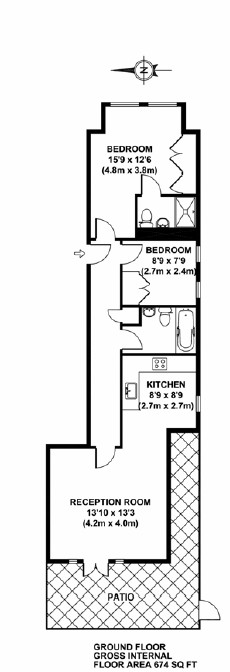This detailed blueprint showcases a compact apartment with a total floor area of 674 square feet. The layout includes two bedrooms: the first features an ensuite bathroom complete with a sink, toilet, and potentially a shower, while the second, adjacent bedroom shares a wall with the first, and has access to a bathroom located down the hall. The arrangement boasts a small kitchen and a reception room, which opens up to a snug patio that wraps around the exterior. A hallway runs along one side, seamlessly connecting all the rooms. Additionally, the blueprint indicates two entrance points: the primary door located to the north and a secondary exit from the patio towards the south, providing versatile access options.